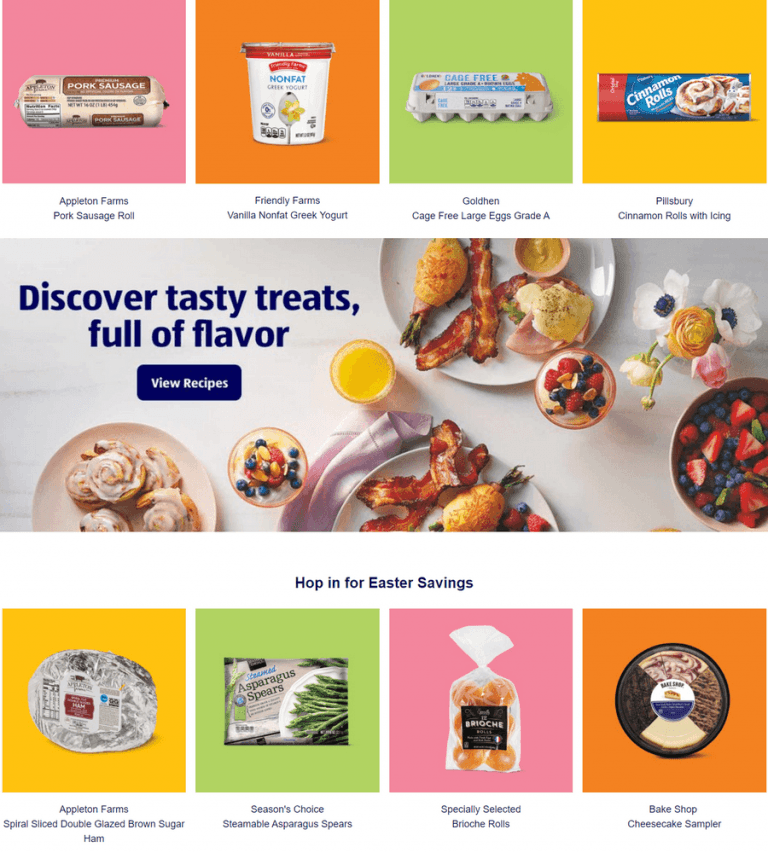The image displays an enticing advertisement centered around a lavish breakfast spread. Dominating the center is a photograph of a beautifully set table adorned with an array of mouthwatering breakfast items. This includes fresh fruits, crispy bacon, golden croissants, and delectable cinnamon rolls. The inviting text atop this image reads, "Discover Tasty Treats Full of Flavor," accompanied by a call-to-action button labeled "View Recipes" beneath it.

The top and bottom of the image are bordered with a collection of vibrant product displays, each set against brightly colored backgrounds in hues of pink, orange, green, and yellow. 

The upper row features:
1. **Appleton Farms Pork Sausage Roll**
2. **Friendly Farms Vanilla Nonfat Greek Yogurt**
3. **Gold Hen Cage-Free Large Grade A Eggs**
4. **Pillsbury Cinnamon Rolls with Icing**

The bottom row highlights:
1. **Appleton Farms Spiral Slice Double Glaze Brown Sugar Ham**
2. **Season's Choice Steamable Asparagus Spears**
3. **Specially Selected Brioche Rolls**
4. **Bake Shop Cheesecake Sampler**

Each product is meticulously showcased with its packaging, ensuring that viewers can easily identify and feel enticed by the offerings.